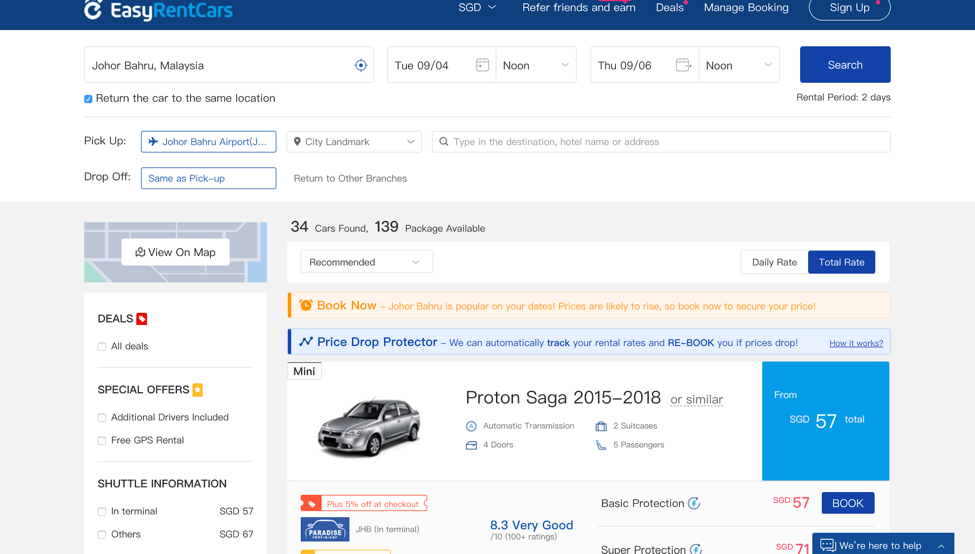The image is a horizontally rectangular screenshot of a section of the EasyRentCars website. It begins with a dark blue horizontal banner at the top. On the left side of this banner is the EasyRentCars logo, and to the right are several options in the following order: a drop-down menu displaying "SGD," a "Refer Friends and Earn" link, a "Deals" section, a "Manage Bookings" option, and a "Sign Up" button.

Below this banner, there is a horizontal row of input fields. These fields allow users to select a rental location, set a check-in date and time, set a check-out date and time for both pickup and drop-off, and click a "Search" button to find rental cars. Beneath these fields, there is information indicating that the location for the drop-off is the same as the pickup location.

Moving further down the image, there is a headline stating "34 cars found, 139 packages available." Due to the partial view of the screenshot, only one car option is fully visible: a Proton Saga from the years 2015 to 2018, with a total rental cost starting from SGD 57.